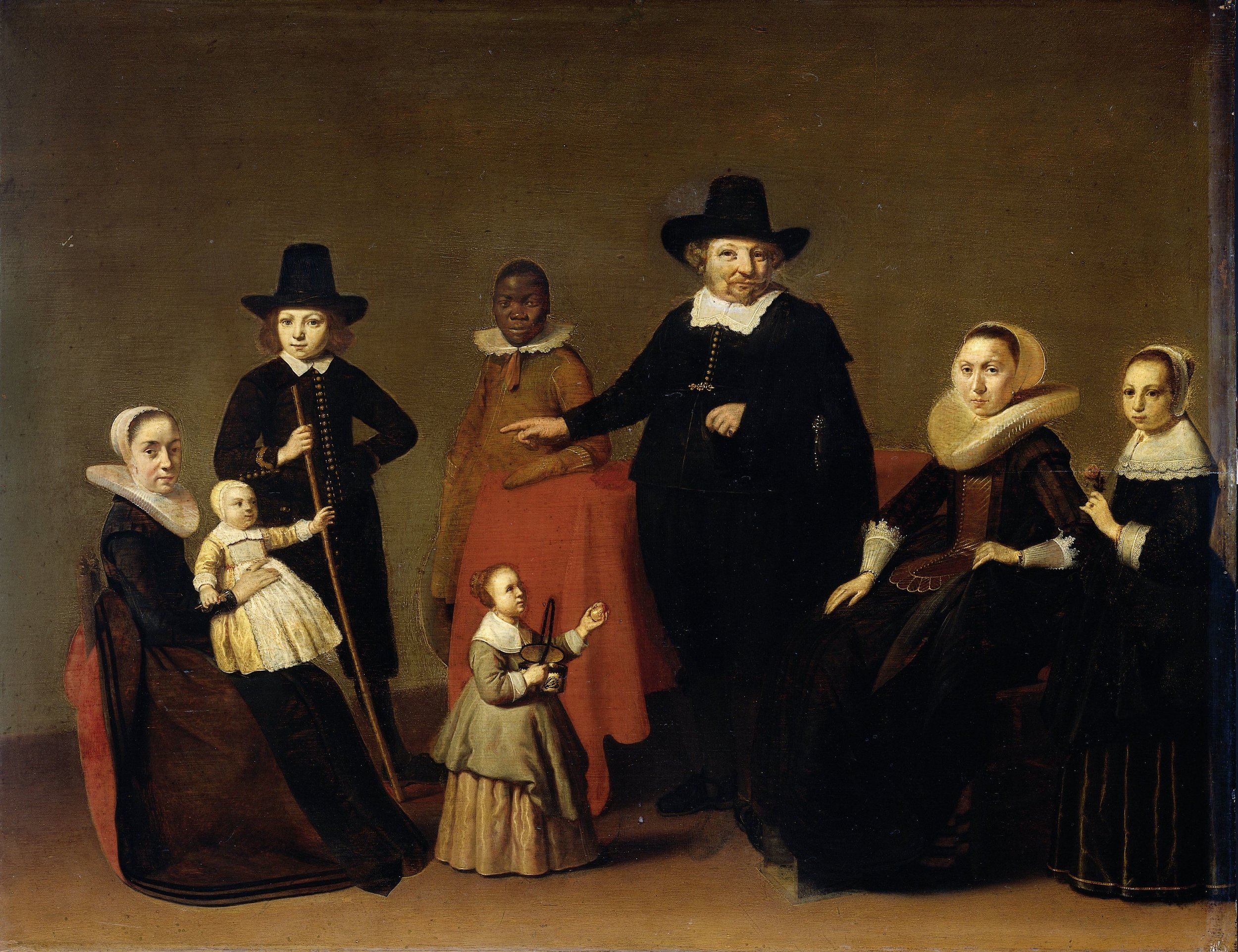This detailed oil painting portrays a group of eight people from the colonial period of America. The scene is dominated by a large group of white individuals predominantly dressed in black. The men, identifiable by their black coats and traditional colonial-style top hats, stand on either side. One man, sporting a small beard, is pointing to his right while looking directly at the viewer. He appears to gesture towards a woman seated on the left who holds a baby. The baby, dressed in white, is juxtaposed by another smaller individual—also in a dress—whose size suggests youth but whose attire mimics an adult's. 

Three white women, all in black dresses adorned with distinctive white collars, flank the scene, adding to the period authenticity. The black hats worn by the men and the bonnets on some of the women enhance the colonial feel of the image. Another unique figure, a black woman in a brown outfit with a similar white collar, stands prominently in the center, providing a striking contrast to the predominantly dark attire. 

The children in the painting stand out for their lighter-colored clothing; a baby in white and a younger child in green who stands with an inquisitive gaze and uplifted hands. The group is assembled in front of a red draped object, possibly a piano, contributing to the painting's complex composition. The background is a muddled blend of brown and olive green hues, adding a sense of depth and mystery to the scene. Overall, this image captures a rich tapestry of colonial life, familial ties, and social dynamics.